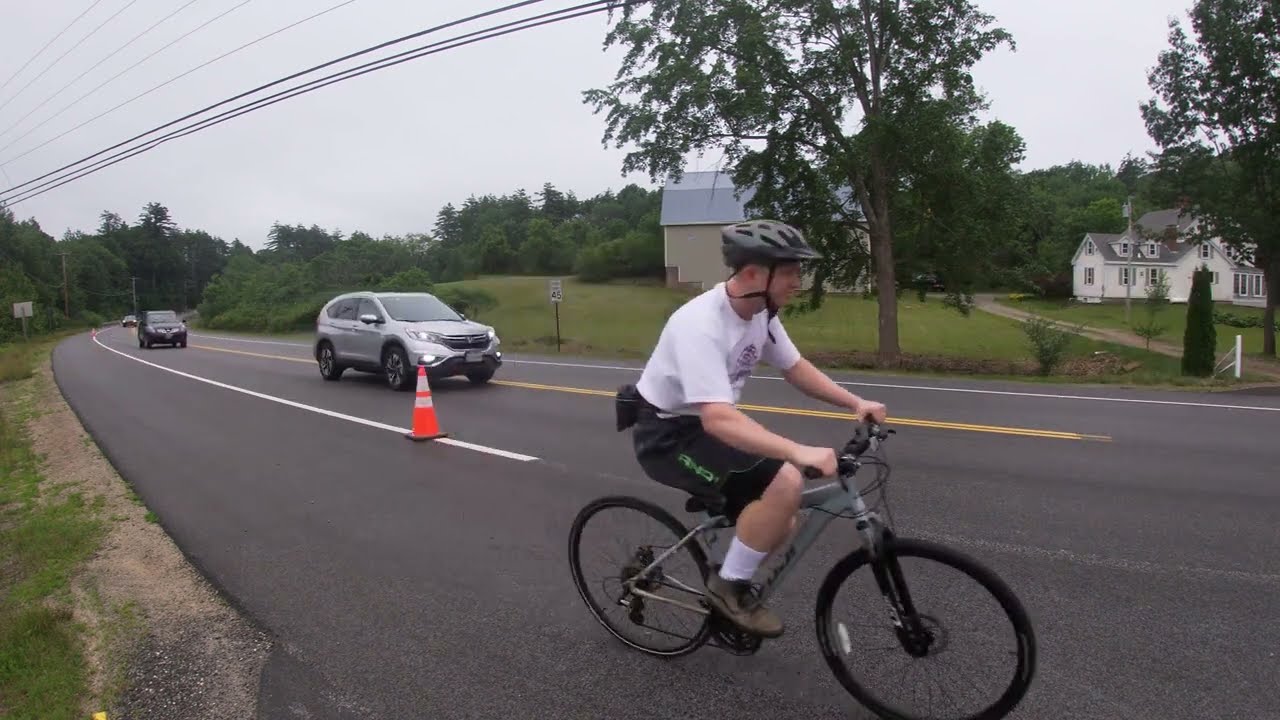This photograph captures a side view of a fair-skinned man cycling on the shoulder of a paved black asphalt road under an overcast sky. He is riding a gray mountain bike adorned with black tires and is dressed in a white short-sleeve t-shirt with a purple design, black shorts, brown shoes, and white socks. A black bicycle helmet rests on his head. The cyclist rides to the right, safely distanced from the vehicles on the road which is marked by a double yellow line and white shoulder lines. 

Adjacent to his path, an orange safety cone is visible before the rider comes into view. Several cars are on the road, including a silver one directly behind the cyclist and another black car further back. The scene is set in a rural area with expansive green fields and tall trees featuring dark green leaves and brown trunks. Across the road, two houses are visible amidst the greenery—a big white house with plenty of windows on the upper right and a tan barn-like structure with a gray curved roof beside it. Power lines cut across the upper left corner of the image. A white road sign on a black post, indicating a speed limit of 45, stands between the cyclist and the distant silver car.